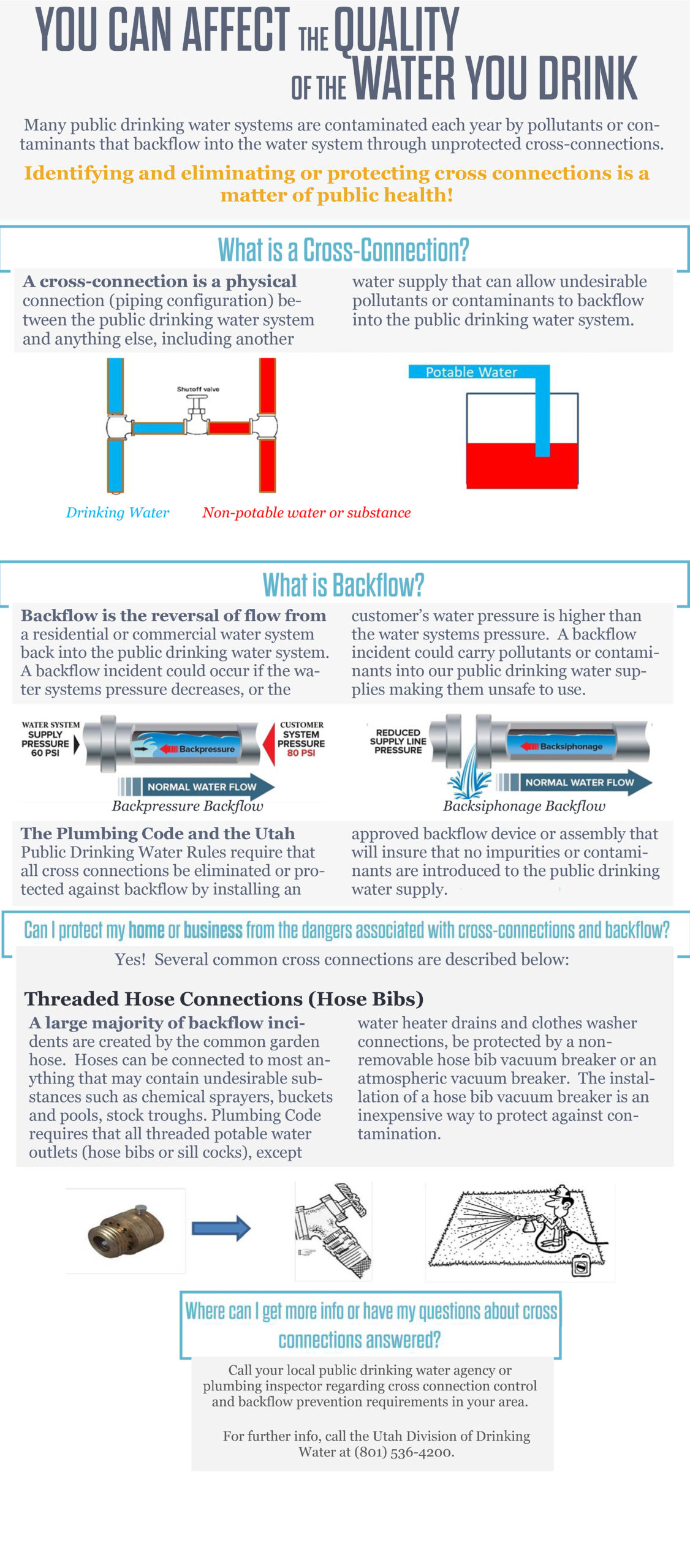This detailed image appears to be a public service poster titled "You Can Affect the Quality of the Water You Drink." It serves as an informational guide on how different qualities of water interact to deliver the best flavor and purity. The content is organized into several distinct sections. The first section, titled "What is a Cross-Connection?", explains how cross-connections occur when a pipe used for potable water links to a pipe carrying non-potable substances, potentially leading to contamination. The second section, "What is Backflow?", describes backflow as the undesirable reversal of flow in a piping system, which can lead contaminants to enter the clean water supply. 

Further, there's another section addressing the question, "Can I Protect My Home and Business from the Dangers Associated with Cross-Connections and Backflow?", providing practical advice on prevention methods. The final section is labeled "Where Can I Get More Info or Have My Questions About Cross-Connections Answered?", directing readers to additional resources. Alongside this information, the poster includes various images of plumbing components, such as valves and pipes in blue and red, to visually illustrate concepts like cross-connections and backflow. This also includes a visual of a man watering grass. Despite the small print, likely making it hard to read all details, the poster aims to educate on protecting public drinking water from contaminants and ensuring water quality.